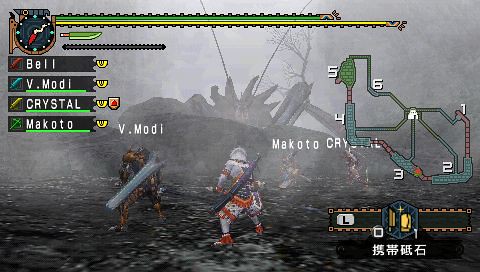The screenshot from this video game captures an intense battle scene set in a post-apocalyptic environment. Various shades of grey dominate the fragmented background, littered with the wreckage of fallen buildings and scattered debris. The terrain appears as a mix of dirt and pebbles in black and grey tones. A HUD with pixelated, retro-style graphics overlays the scene, providing crucial game information. At the top, green and yellow progress bars are displayed, alongside a time clock situated in the top left corner.

Four names are listed prominently: Bell, V-Mody, Crystal, and Makoto. These likely correspond to key players or characters involved in the action. Two central figures are engaged in combat: one wielding a long knife and the other brandishing a large metallic weapon. A menacing, large insect-like creature looms in the background, hinting at the adversaries they face. 

Additional text elements include Chinese or Japanese kanji characters positioned at the bottom right, and a numbered map labeled 1 through 6, indicating player locations in the game. One character, dressed in silver and red and possibly armed with a rifle, stands prominently in the scene, embodying the player’s avatar amidst the chaotic battle.